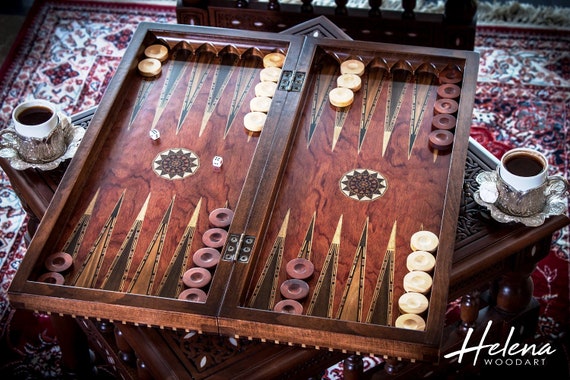This photograph features an exquisite, elite backgammon set crafted from beautiful mahogany wood, complemented by intricately carved black wood design on its inner section. The set is elegantly positioned diagonally on an ornate wooden cocktail table to make space for two white mugs with chrome accents, placed in fancy silver holders adjacent to the game, evidently for the convenience of the players. These elements rest atop a luxurious red, cream, and dark blue oriental rug adorned with intricate patterns, including hearts and diamonds. The image captures a moment seemingly set for an anticipated game, evidenced by the positioning of game pieces suggesting arrangement for play, and the overall setting exudes a sense of opulence and sophistication. At the bottom of the picture, the words "Helena Wood Art" subtly affirm the origin of this masterfully crafted set.